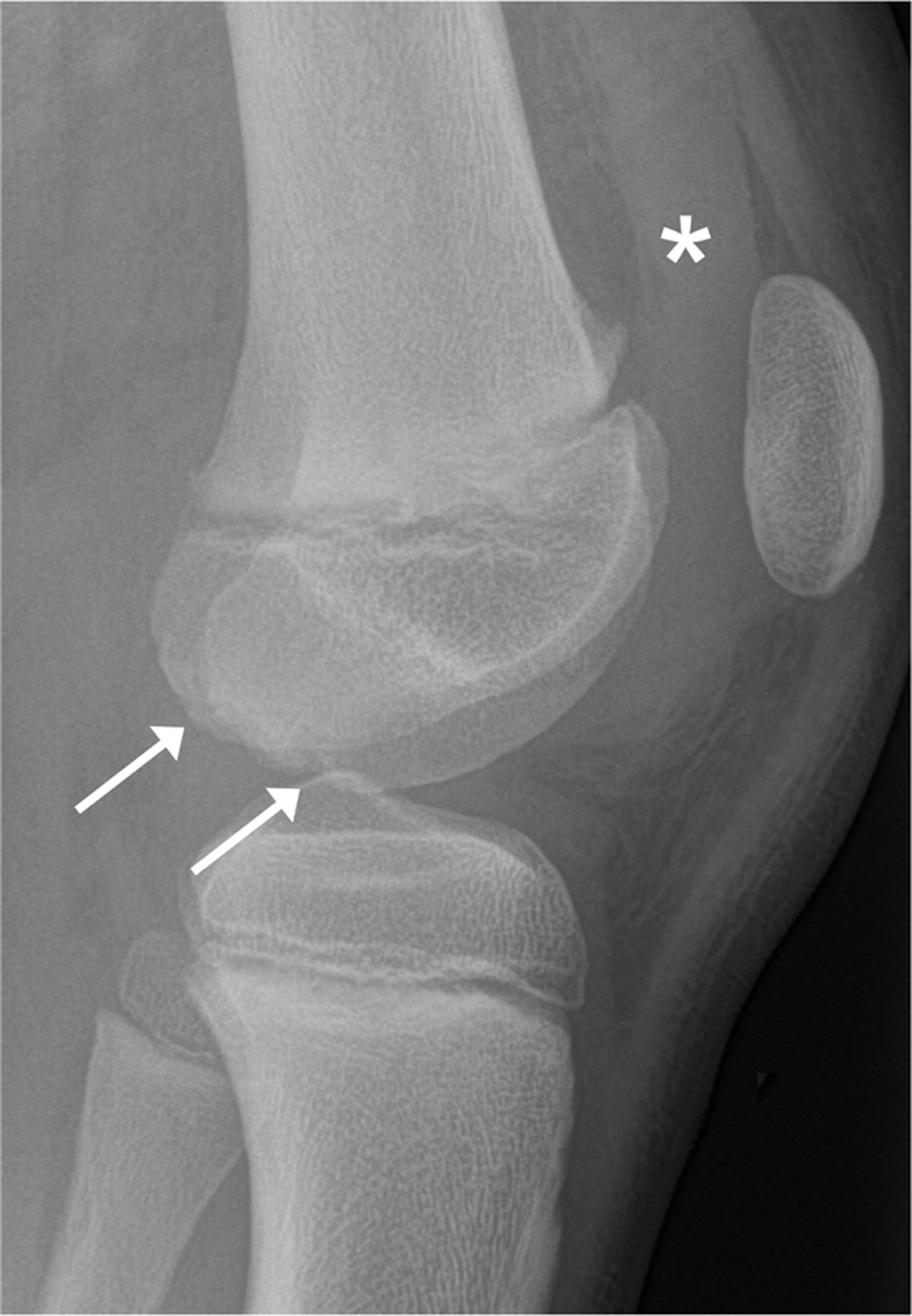This image is a detailed black-and-white x-ray showing the hip and leg bones. The primary focus appears to be on the junction where the ball and socket of the hip meet. The x-ray highlights these areas with two white arrows, possibly indicating a break or disconnection in the bones. Additionally, there's a white asterisk near the hip bone, which might denote another area of interest or concern. The photograph also shows a small mass to the right of the main bones, which is not a bone but might be relevant to the diagnosis. The overall x-ray provides a clear view of the bone structure, with the typical grayscale coloration distinguishing bone density and soft tissue variation.